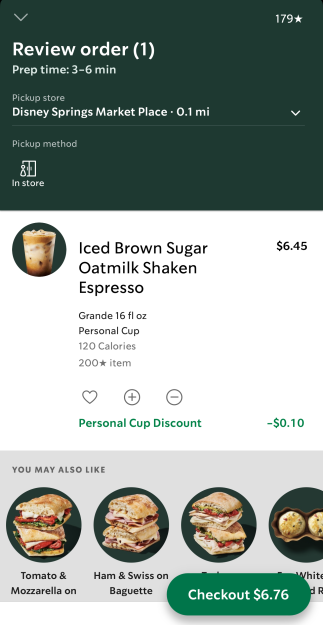A detailed caption for the screenshot of the ordering app:

"This screenshot from the Starbucks ordering app captures the 'Review Order' screen in detail. The upper third of the screen features a dark green background with white text. In the top-left corner, there's a drop-down arrow, and on the right, it displays '179 stars.' Prominently in the center, bold text reads 'Review Order (1),' beneath which the prep time is listed as ‘3-6 minutes.’ The designated pickup location is 'Disney Springs Marketplace,' located 0.1 miles away, with options to select or change this store. The pickup method is specified as 'In-store.'

Highlighted in the order details is a 'Brown Sugar Oat Milk Shaken Espresso' drink. An icon to the left shows an image of the drink. The description notes it as 'Grande, 16 fluid ounce, personal cup, 120 calories, 200-star item,' priced at $6.45. Below the item, there is a heart icon, a plus-minus button for quantity adjustment, and green text indicating a 'Personal Cup Discount' of 10 cents.

At the bottom, a gray bar provides suggested food items labeled 'You May Also Like,' featuring options such as 'Tomato and Mozzarella,' 'Ham and Swiss on Baguettes,' alongside other partially obscured items. The screen concludes with an oblong green 'Checkout' button displaying a total amount of '$6.76.'"